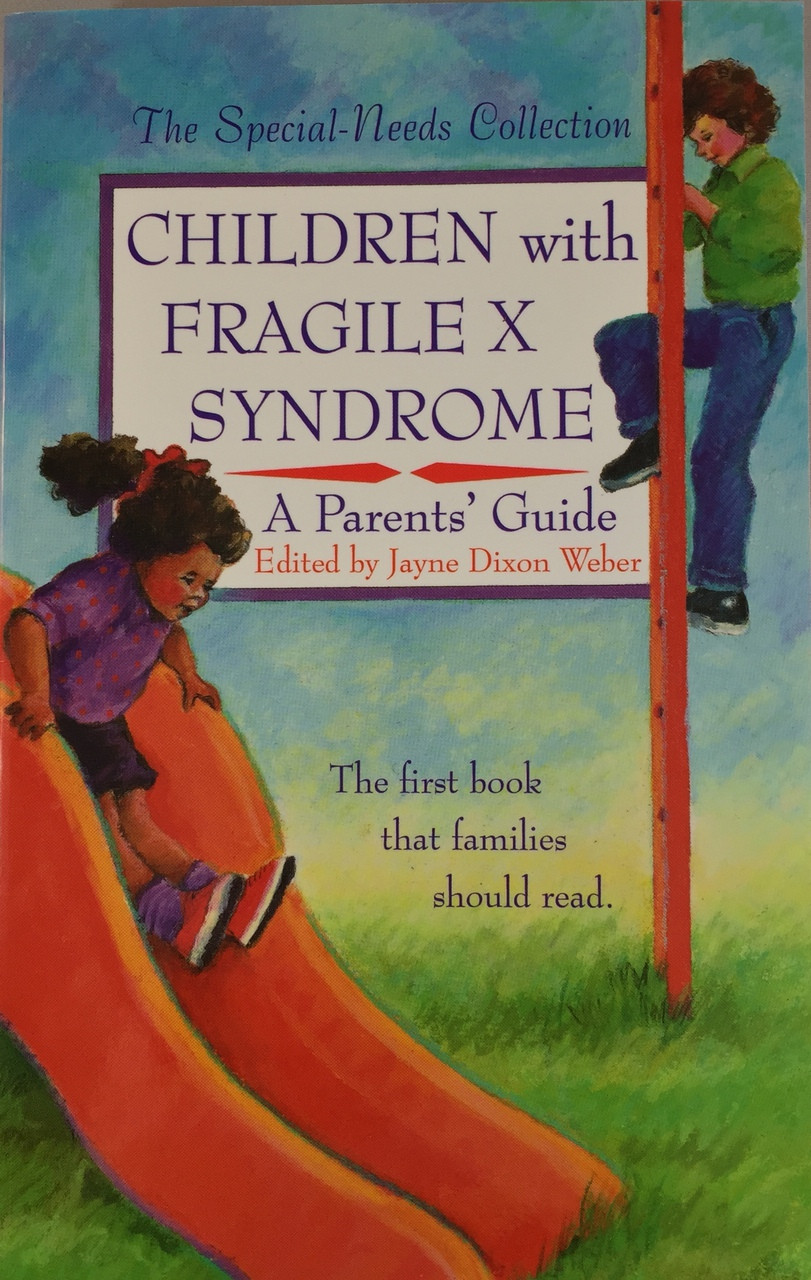The cover of the book "Children with Fragile X Syndrome: A Parent's Guide" edited by Jane Dixon Weber, features vibrant artwork primarily with shades of blue and green. The scene depicts a young boy, around eight years old, dressed in jeans and a green shirt, climbing an orange pole that extends off the cover. To his left, a girl, approximately five years old with brown curly hair and a red bow, slides down a dark orange slide. The ground beneath them is a lush green, evoking grass. The title and various details of the book are presented in a white box outlined in purple, with the text in complementary shades of purple and orange. This book is part of "The Special Needs Collection" and is recommended as the first book families should read. The cover, illustrated with what appear to be markers or colored pencils, exudes a welcoming and informative visual appeal.